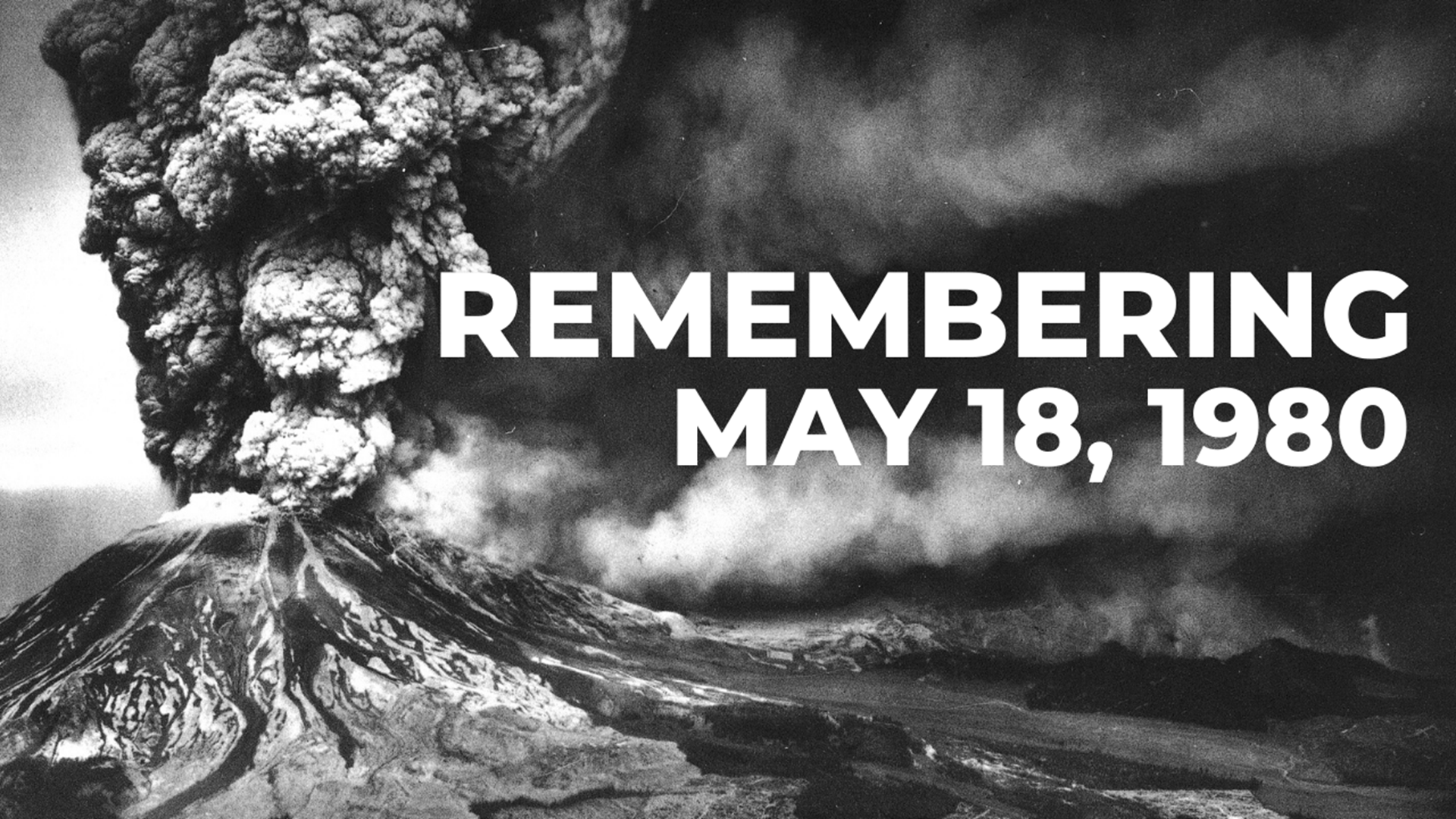This striking black-and-white photograph captures the dramatic eruption of a volcano on May 18, 1980. The massive plumes of smoke and ash billow relentlessly from the left side of the volcano, creating an immense, billowing cloud that darkens the right side of the sky. Hot, molten lava floods the valley below, pouring out from the mountain's peak in a relentless and terrifying flow. The eruption's intensity is starkly accentuated by the thick, dark clouds filling the sky, suggesting the airborne ash's extensive spread. The image is overlaid with a bold, white caption in all capital letters, centrally placed on the right side, which reads, "REMEMBERING May 18, 1980," drawing attention to this historic and catastrophic event.